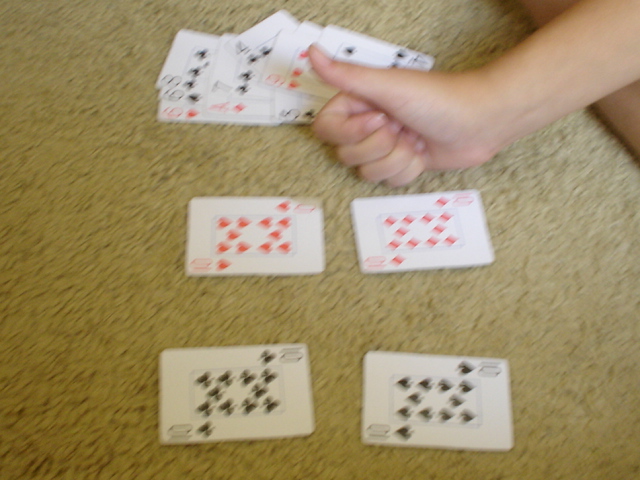The photograph appears blurry but captures a scene where an individual is seated on an old, worn, brown carpeted surface. Partial views of their leg and hand are visible. The person's hand, giving a thumbs up, is located next to an arrangement of playing cards spread out on the carpet. Among the cards, four white cards numbered 10 (10 of hearts, 10 of diamonds, 10 of spades, 10 of clubs) are distinctly visible, representing both black and red suits. To the right of the hand is a disorganized stack of additional cards showing numbers such as 6, 6, 8, 7, 4, 3, 9, and 4 across various suits including hearts, spades, and clubs. The environment appears dimly lit, contributing to the overall darkness and lack of clarity in the image.